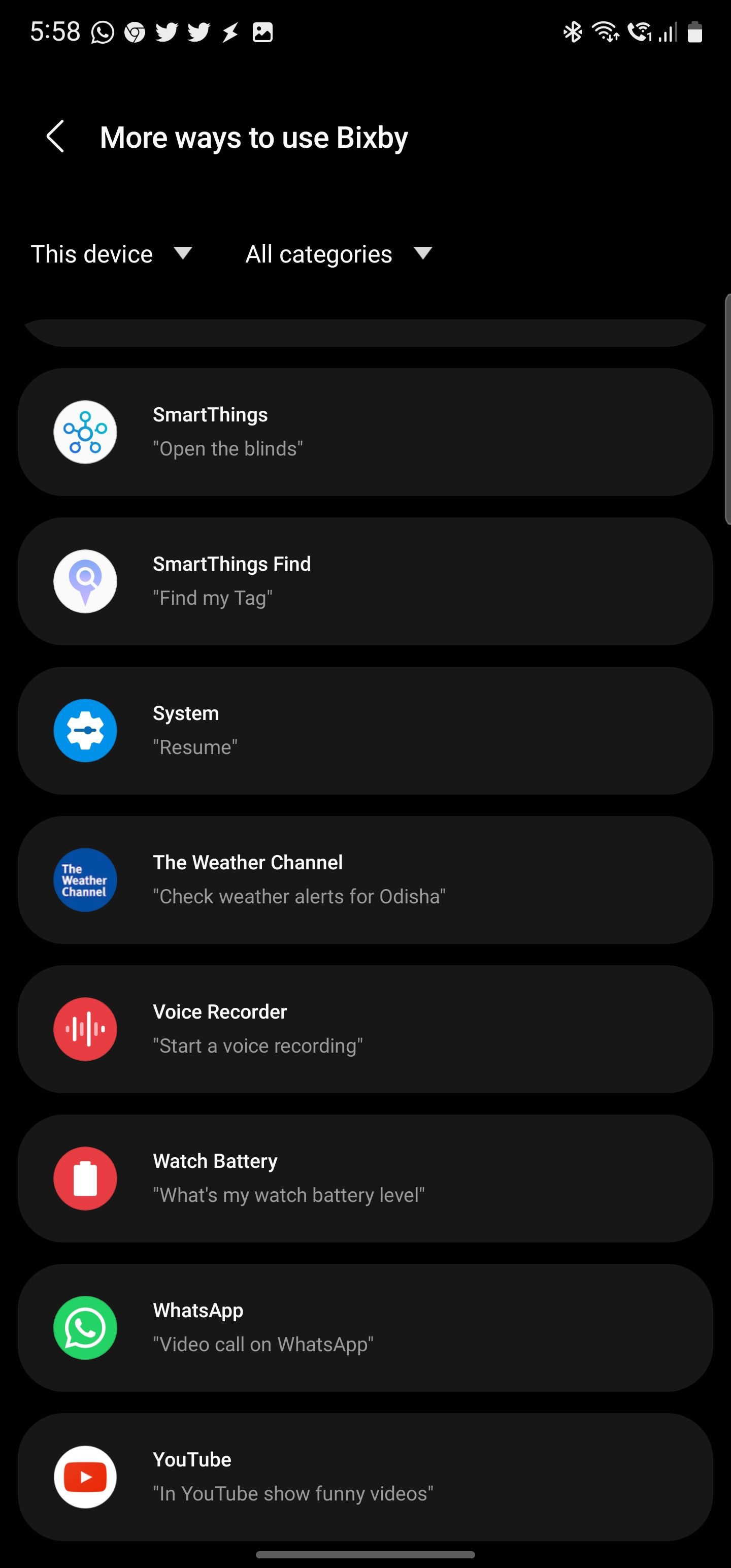A detailed screenshot of a smartphone screen displaying the "More ways to use Bixby" page is open within the settings category. The background is black with vibrant icons in primary and secondary colors for various applications and settings, including SmartThings, SmartThings Find, System, The Weather Channel, Voice Recorder, Watch, Battery, WhatsApp, and YouTube. The top of the screen shows a black banner indicating the user is browsing in Chrome. It is 5:58 PM, and visible are two Twitter icons and an indistinct lightning bolt symbol. The settings menu highlights options for Bluetooth and Wi-Fi.